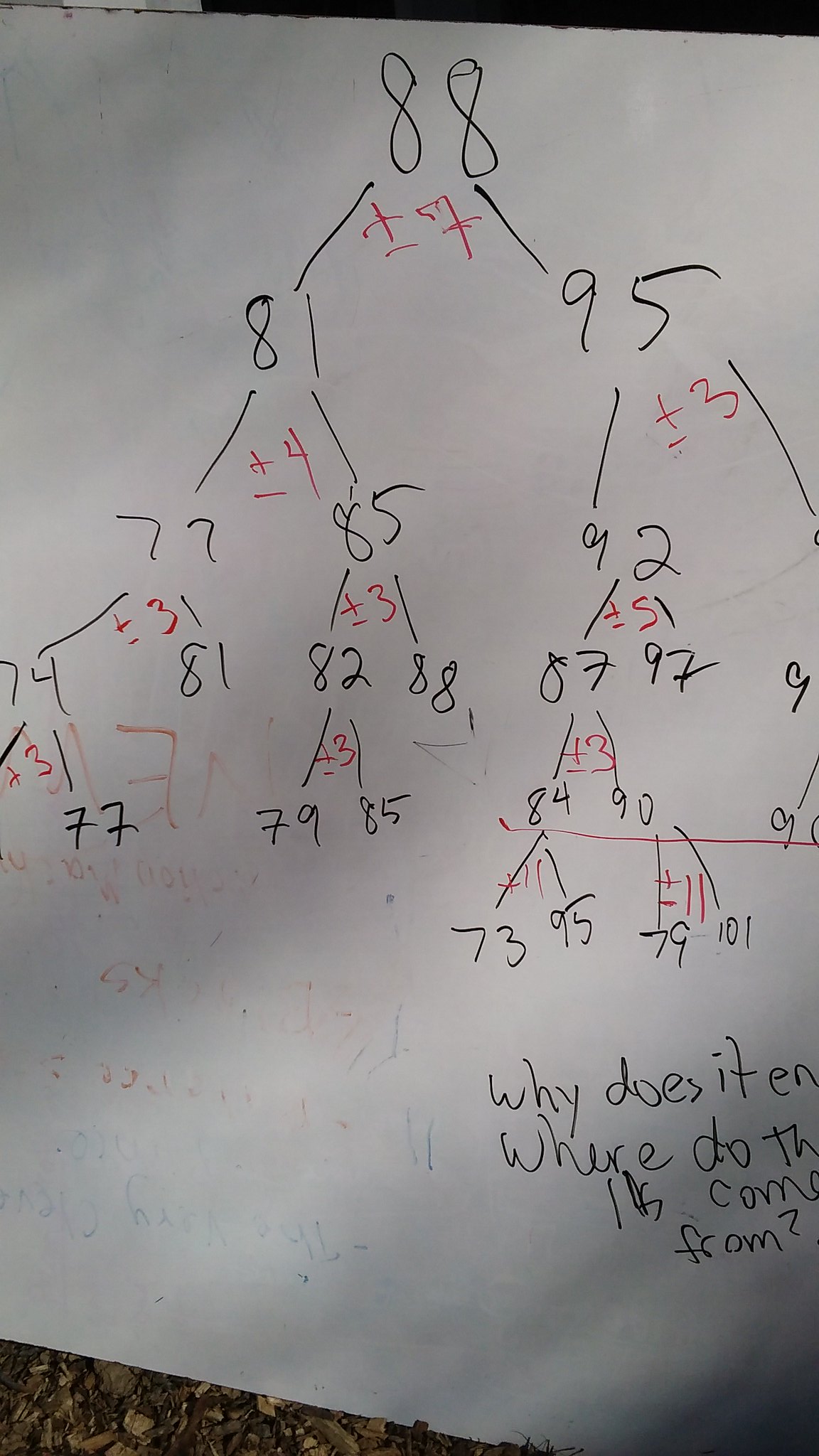In the photograph, there is a mathematical diagram drawn on a whiteboard. At the top of the diagram, the number "88" is prominently written in black marker. From this number, two diagonal lines extend outward to the sides.

Directly beneath the "88" is the notation "±7" written in red. The left diagonal line leads to the number "81," which also has "±4" written beneath it in red. This "81" then branches into two more numbers, "77" and "85." Both of these numbers have "±3" written underneath them in red and further branch out.

The number "77" splits into "74" and "81," with both of these numbers having "±3" written in red beneath them. The number "74" also extends into two more lines, but the left number is cut off. The right number is "77." Similarly, the "82" branches into "79" and "85," each with diagonal lines extending out.

Returning to the original "88," the right diagonal line leads to the number "95," which similarly splits into two lines below. Underneath "95," we see "±3" written in red. The writing on the right is cut off, but the left line leads to "92," which has "±5" written beneath it in red. This "92" then branches into "87" and "97."

The number "87" further splits and has "±3" written beneath it in red, extending into "84" and "90." Each of these numbers has "±11" written in red, and they then branch further into "73, 95" from "84," and "79, 101" from "90."

Overall, the diagram showcases a complex hierarchical structure of numbers with associated plus or minus values, all meticulously laid out in black and red marker on the whiteboard.